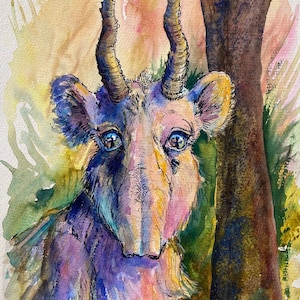The image is a colorful painting or illustration of a fantastical creature that resembles an anteater or a distorted elephant. The creature is painted in a medley of colors, including blue, orange, green, pink, and other vivid hues, creating a visually striking appearance. It has two large, glossy eyes that give it an expressive look. Its nose is notably long and wide, resembling a double-barreled trunk, and leads down to its mouth area. Crowning its head are two curvy, tan-colored horns that protrude from the top of its forehead. The ears are relatively large and round, positioned on the upper sides of its head.

The background of the painting includes various natural elements. To the right of the creature, there's a prominent dark brown tree trunk or stump, alongside green blobs representing foliage. There are also yellow, gray, and reddish plants or stems scattered throughout the background, adding depth and complexity to the scene. The creature's body, visible up to the shoulders, is painted in a combination of blue, yellow, pink, and purple, contributing to the overall vibrant and fantastical atmosphere of the artwork.